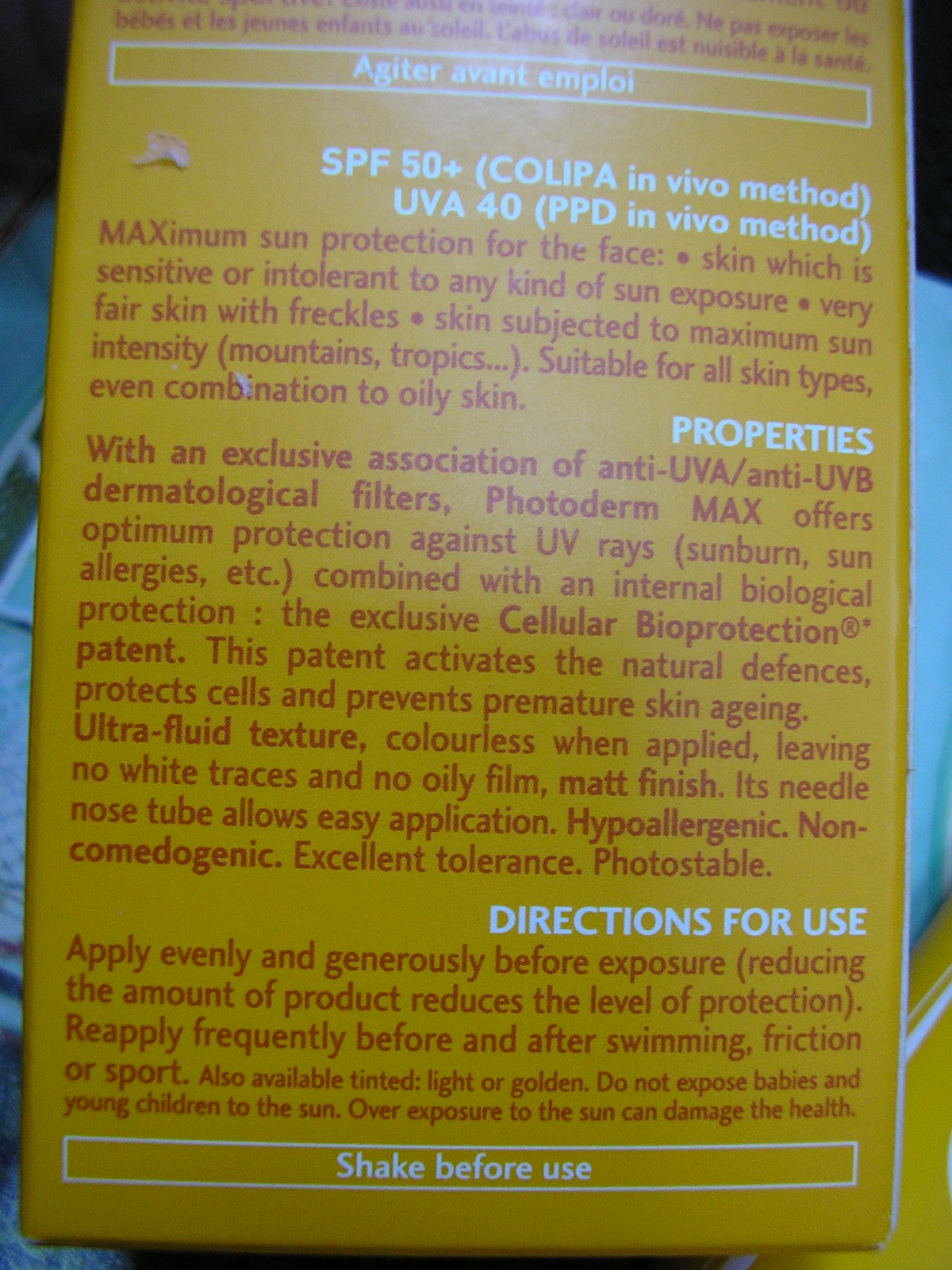**Caption:**

The image features the side of sunscreen packaging, labeled with SPF 50+ and UVA 40, indicating maximum sun protection. It's designed for the face and suitable for those with sensitive, intolerant skin, very fair skin with freckles, and skin exposed to intense sun conditions like mountains or tropical regions. It is appropriate for all skin types, including combination to oily skin. The packaging highlights several key properties:

- **Dermatological Filters:** Combines anti-UVA and anti-UVB filters for optimum protection against UV rays, sunburn, sun allergies, etc.
- **Biological Protection:** Features an exclusive Cellular Bioprotection® patent, which activates natural defenses, protects cells, and prevents premature skin aging.
- **Texture and Finish:** Ultra-fluid, colorless when applied, leaving no white traces and no oily film, with a matte finish.
- **Application:** Its needle-nose tube design ensures easy application. 
- **Formula:** Hypoallergenic, non-comedogenic, excellent tolerance, and photo-stable.

**Usage Directions:**
Apply evenly and generously before sun exposure. Reducing the amount of product used lowers protection. Reapply frequently, especially after swimming, friction, or sports activities. Also available in tinted versions: light or golden. Always shake before use.

**Safety Warnings:**
Do not expose babies and young children to the sun. Overexposure to the sun can be harmful to their health.